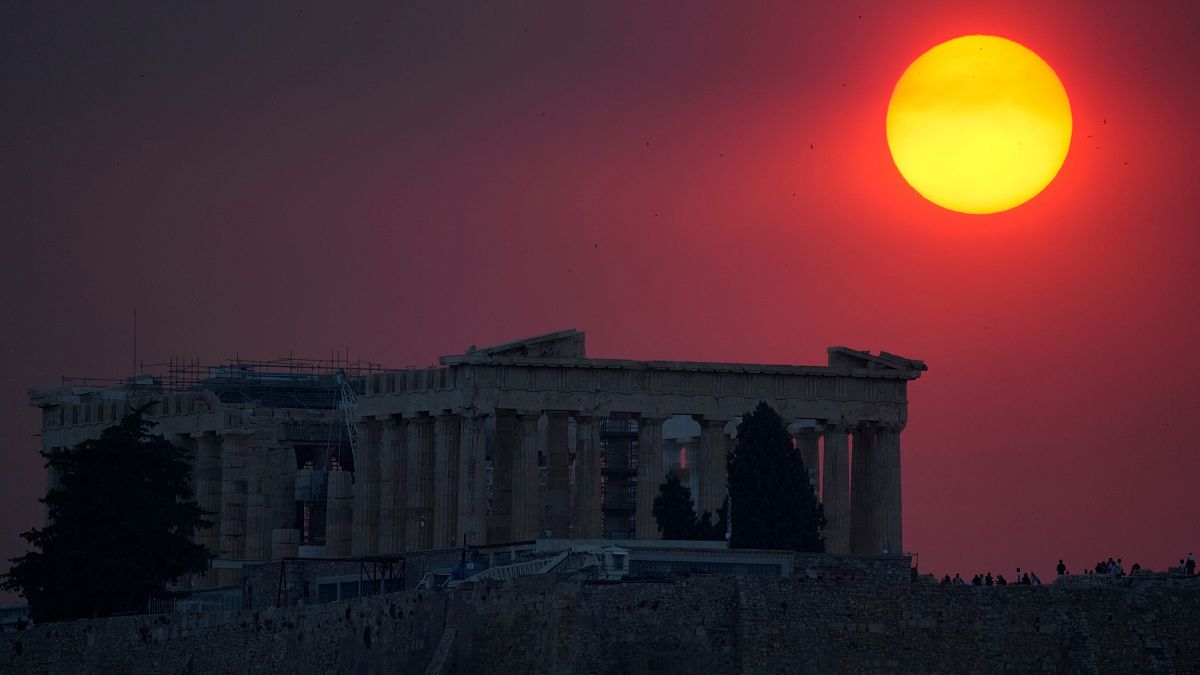This nighttime outdoor image features an ancient, castle-like structure silhouetted against a dramatic, color-filtered sky. The building, possibly the ruins of the Parthenon or a similar classical structure, appears dimly lit, with multiple columns and archways barely visible. The structure's flat roof is adorned with apparent scaffolding and construction equipment, indicative of ongoing restoration work. In front of the building, three evergreen trees stand in silhouette. The backdrop boasts a striking sky that transitions from a deep crimson color to almost black on the left side. Dominating the top right corner is an intensely bright, lemon-orange moon surrounded by a fiery orange ring, casting a surreal glow over the landscape. The sky beneath this celestial body displays hues of deep red and purplish tones, enhancing the ethereal atmosphere. The image's detailed composition combines photographic realism with special effects, adding to its profound visual impact.